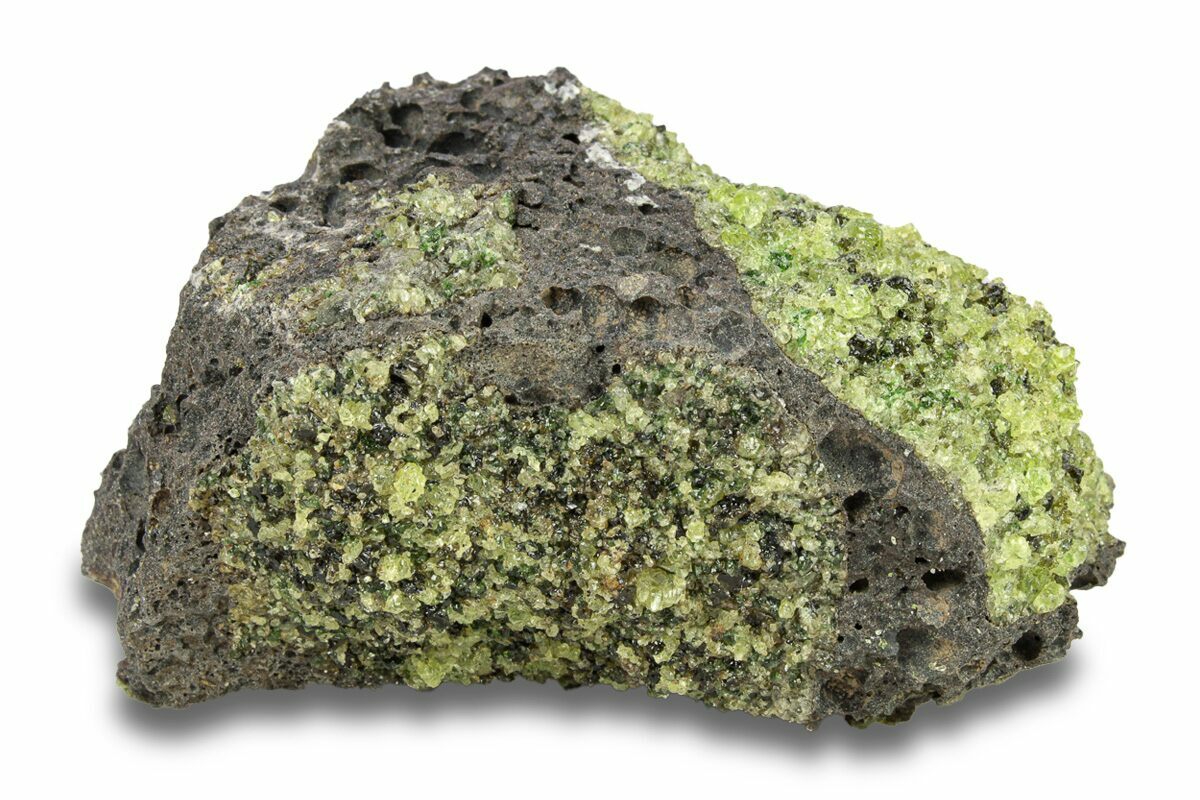This color photograph, taken in landscape orientation, features a close-up view of a uniquely shaped mineral or rock resting on a white surface. The rock is wider than it is long, with an irregular form that’s broader on the left and tapered towards the right, resembling an elongated, somewhat oval shape. The base of the rock is a pitted, dark gray color, interspersed with large holes and a very textured surface, especially prominent on the upper left section. This gray material extends in a stripe-like pattern from the upper left to the bottom right. Covering much of the rock are clusters of light green, translucent crystals, which form a striking contrast against the darker base. These green crystals are especially concentrated in the center and right side of the rock, creating a patchy appearance where the light lime to mint green crystals dominate the surface. The rock casts a subtle shadow on the white background, indicating it is lit from above.